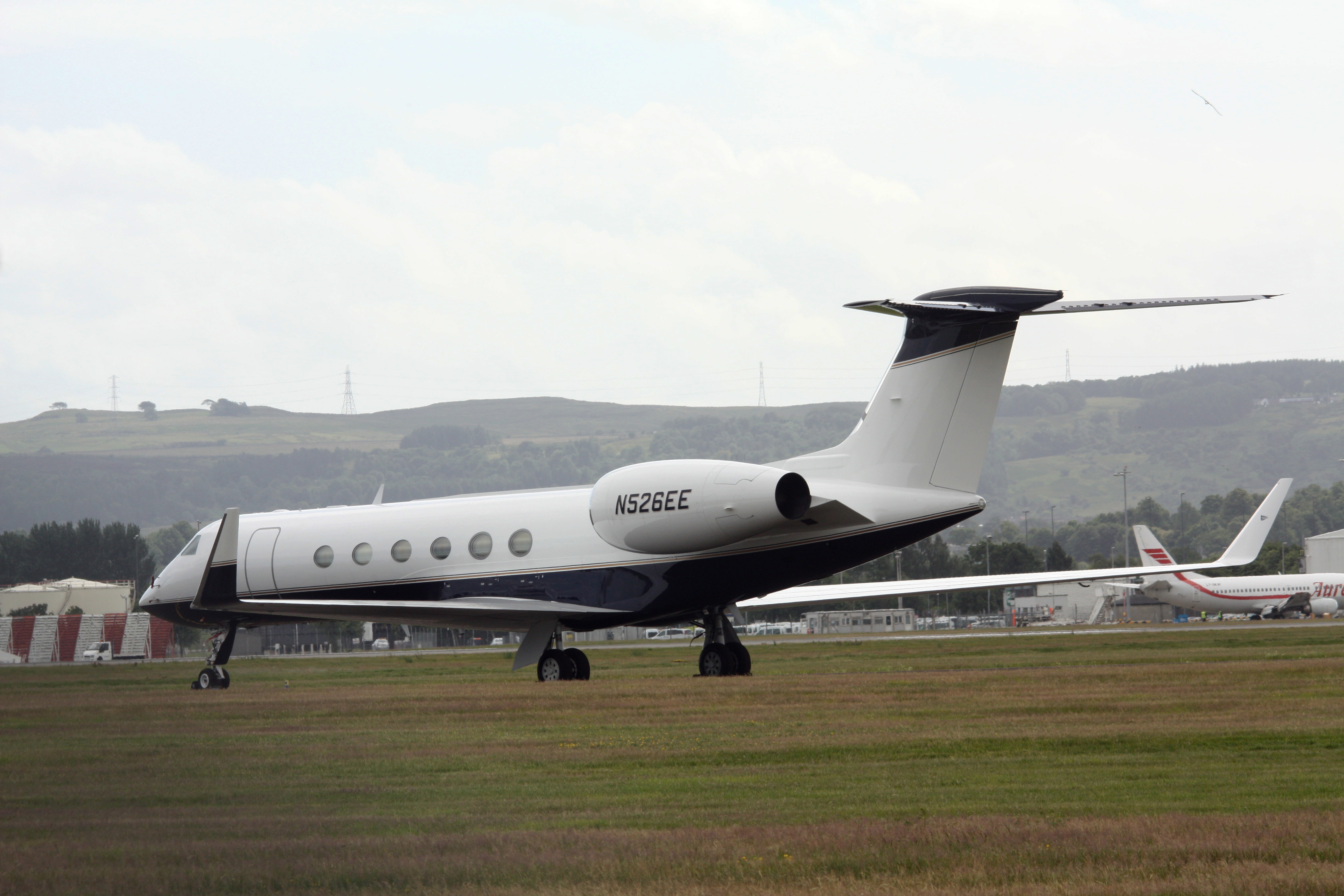This landscape-oriented color photograph features a private jet, prominently positioned in the center, with the registration number N526EE visible on its rear engine. The jet is a sleek combination of white, grey, and blue, with six round windows dotting its side. It is parked on a grassy area, with the grass appearing predominantly green with some gold patches. 

Behind the private jet, there is a bustling airport scene, including an official commercial airplane, possibly a Boeing 737, hinting at the facility's regular traffic. The background is characterized by a low, dark green mountain range adorned with utility poles and power lines, creating a dynamic contrast with the sky. The sky itself is a mix of blue and clouds, indicating fair weather, with a solitary seagull visible in flight. Additionally, there is a small building to the left of the jet, adding to the realism and depth of the scene. 

Overall, the photograph captures a juxtaposition of the tranquil private jet against the busy, structured environment of an airport, encapsulated in a photographic representationalism style.